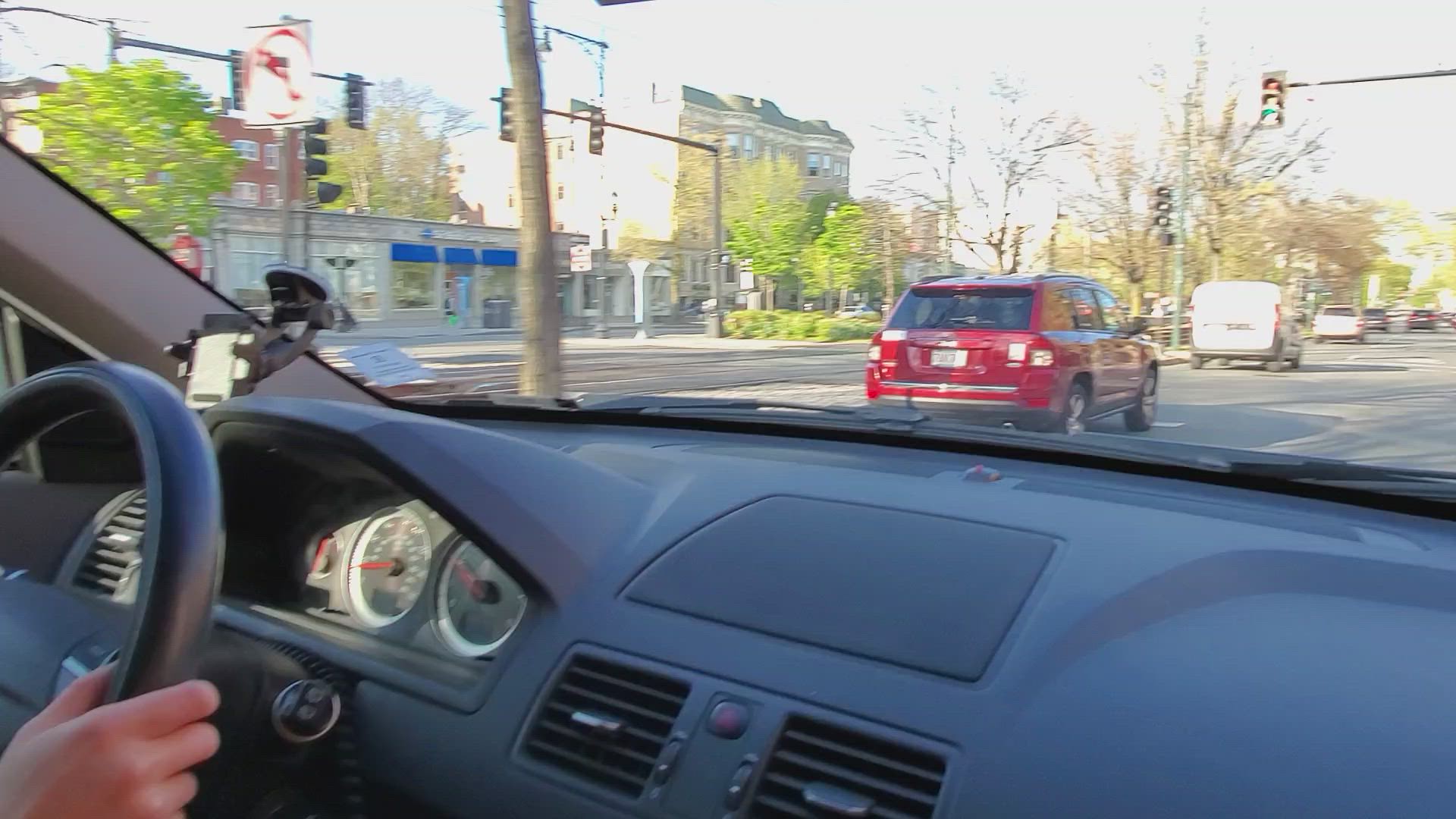Captured from the passenger seat inside a vehicle, this daytime photograph features various details. Within the car, notable elements include a black dashboard equipped with air vents and a steering wheel. There is also a visible hand, presumably the driver's, and a cell phone mount affixed to the windshield.

Visible through the windshield is an urban scene. Directly ahead, a red van and a white van are stopped at a traffic light, which hangs overhead. Additional stoplights are seen on a nearby side street. A green leafy tree is prominently visible in front of the car, set against a backdrop of both verdant and barren trees. To the side, a collection of buildings can be seen, including red brick structures, a tan building, and a squat tan building with a blue awning. Near the leafy tree, a red and white stop sign is also noticeable, adding to the urban landscape.